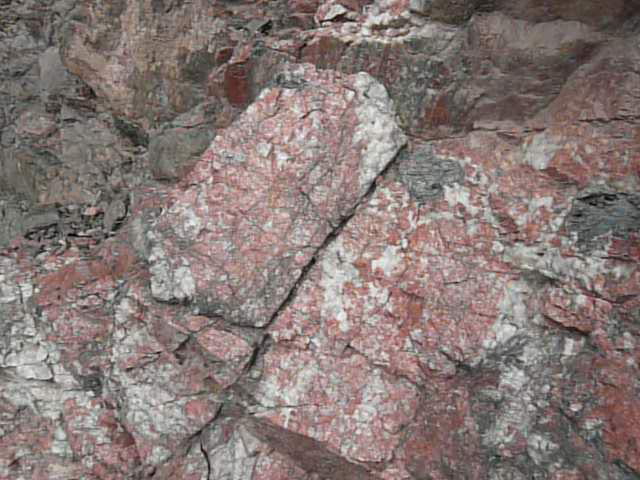This image is a detailed top-down view of a rocky, arid landscape featuring a predominantly red rock formation interspersed with specks of grey and white. The central region of the image showcases the red rocks, which appear to be chipped and eroded, likely from natural wear or external disturbance. Small pebbles matching the larger rocks in color—red, dark grey, light grey, and white—are scattered primarily on the left side of the photograph. The left and top-left corners of the image reveal a lower area, with rocks seemingly piled higher towards the center and right, creating a stepped appearance. The rocks in the top-left corner are noticeably more jagged and textured. The overall scene hints at an outdoor setting, possibly off the side of a cliff or in a dry, cave-like environment. The photo's quality is slightly unfocused, and some rocks display a tan hue, especially towards the top left.